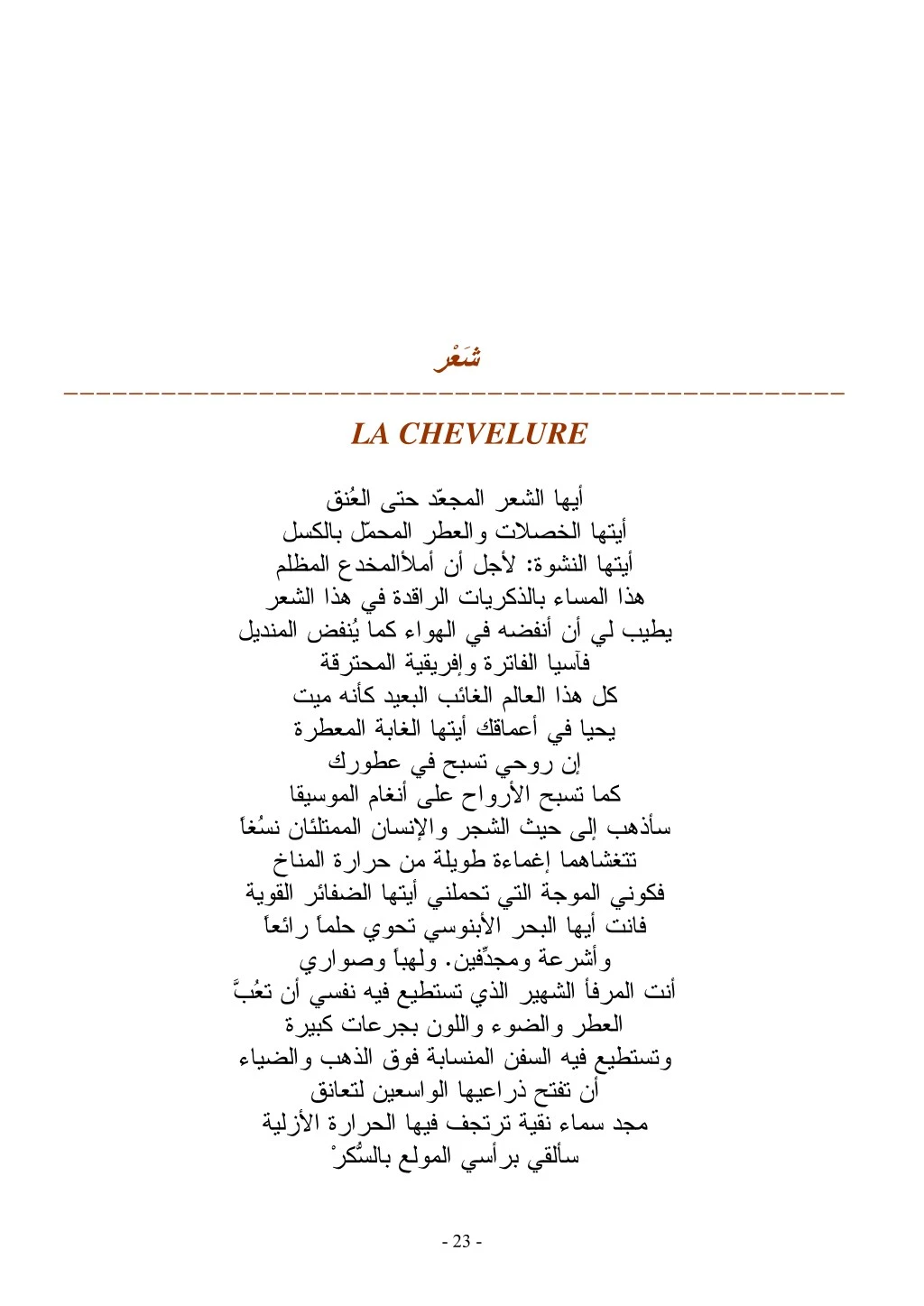The image features a stark white background with an intricate design predominantly utilizing text elements. At the very top, written in a presumably Middle Eastern script resembling Arabic calligraphy, is brown text that seems ornamental or indicative of a title. Directly below this, a dashed line extends horizontally, accentuating the transition between sections of the image.

Centered beneath the dashed line is the phrase "La Chevelure" in a capitalized format, written in brown text and standing out prominently. This translates to "The Hair" in English. Following this title are approximately 20 centered lines of script, characterized by jagged, curvy, and straight lines, likely in the same Middle Eastern language as the initial text.

Finally, at the bottom-right corner of the image, the faded number "23" can be discerned, possibly indicating a page number. This setup with the uniform alignment and the detailed script gives the feel of a poetic or literary excerpt, potentially from a digital book or a scanned ancient manuscript.